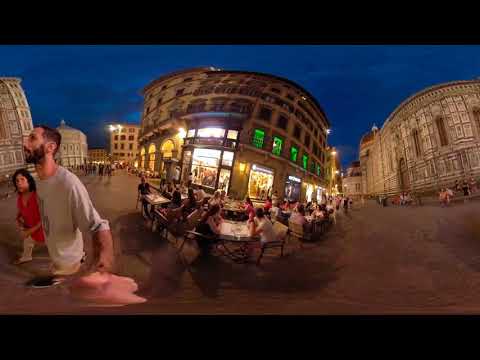The panoramic, fisheye-lens photograph captures a bustling city square at dusk. The sky is a darkening blue, contrasting with the warm, bright lights from the buildings that illuminate the scene. Dominating the center of the image is what appears to be a rounded cathedral or café. The main building has a large window in front, topped with four smaller windows emitting a greenish glow. In front of the building, tables adorned with white tablecloths are fully occupied by people, adding to the lively ambiance. To the left side of the image, a couple is seen walking. The man, dressed in a grey shirt and sporting a beard, looks upwards while holding something pink in his hand. Beside him, a woman with dark hair wears a red shirt and white pants, glancing towards the camera. On the right side of the photograph, people are either passing by or lounging on stair steps leading up to the main building. The streets extend on both sides of the square, with more people walking and mingling, completing the vibrant urban night scene.